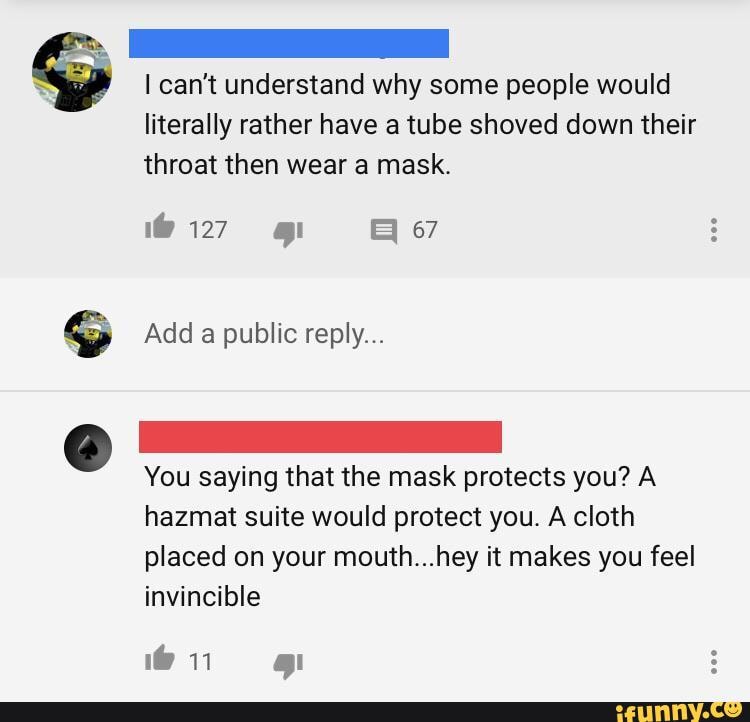The image is a slightly taller-than-wide square depicting a gray-backgrounded thread from what appears to be a social media or forum platform, likely mimicking the YouTube comment format.

At the top-left of the image, there is a comment with a profile picture featuring a Lego man dressed in a sailor outfit with his arms raised, seemingly yelling. The profile name is obscured by a horizontal blue rectangle at the top-right of the comment. The comment text, in black font, reads: "I can't understand why some people would literally rather have a tube shoved down their throat than wear a mask." Below this text, the comment has received 127 thumbs up, with no visible downvotes, and has garnered 67 comments. 

Beneath this, the same profile picture appears, albeit smaller, with the prompt "add public reply..." indicating where users can type a response.

Further down, another profile picture, this time an image of a spade, accompanies a second comment where the user's name is also blocked out. The comment responds to the mask debate, stating: "You saying that the mask protects you, a hazmat suit would protect you, a cloth placed on your mouth. Hey, it makes you feel invincible."

The image captures a snapshot of the ongoing discourse on mask usage, with the upper comment expressing confusion about mask resistance and the lower comment questioning the effectiveness of masks by comparing them to hazmat suits.